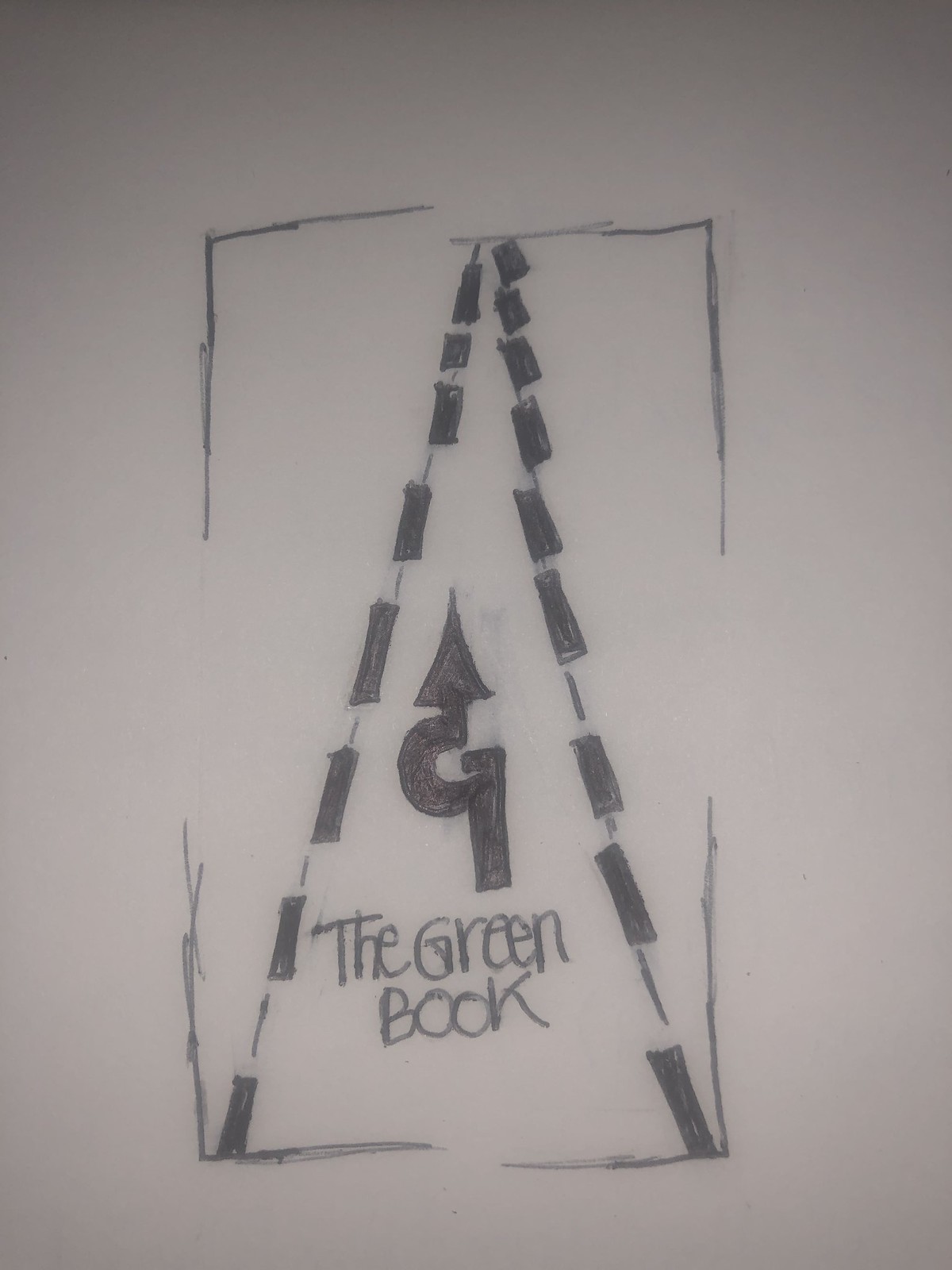The image is an ink drawing on a grayish-white background, likely meant for a book illustration. The rectangular drawing features black-lined sketches and blocks filled with black, resembling a road narrowing towards the top, forming a triangle akin to a Christmas tree shape. Centered within this configuration, handwritten in dark pencil, are the words "The Green Book." An arrow, also dark-colored and curved before becoming straight, points upward towards this text. The overall background is a grayish-white tone, reminiscent of a slightly shadowed room, emphasizing the hand-drawn details of the image.